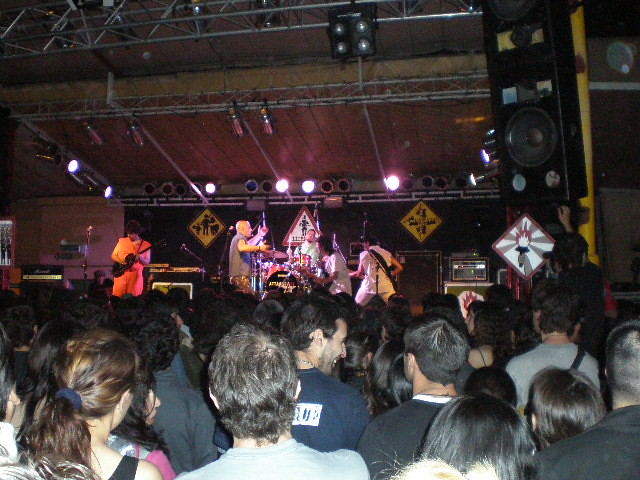This photograph captures a live outdoor concert with a band performing on a stage covered by silver scaffolding and a black tarp acting as a roof. Multiple spotlights hang from the scaffolding, illuminating the band below. In the foreground, the backs of audience members’ heads are visible as they enthusiastically watch the performance. On the right, a large rectangular speaker hangs from yellow scaffolding. The stage hosts five bandmates, including a drummer seated behind black and red drums at the center. On the far left, one band member, wearing an orange sleeveless tank top and matching orange pants, stands out with a spiky black wig and a black electric guitar. The overall scene is dimly lit, creating a dynamic yet dark atmosphere, with the striking orange attire of the guitarist providing a vivid contrast.